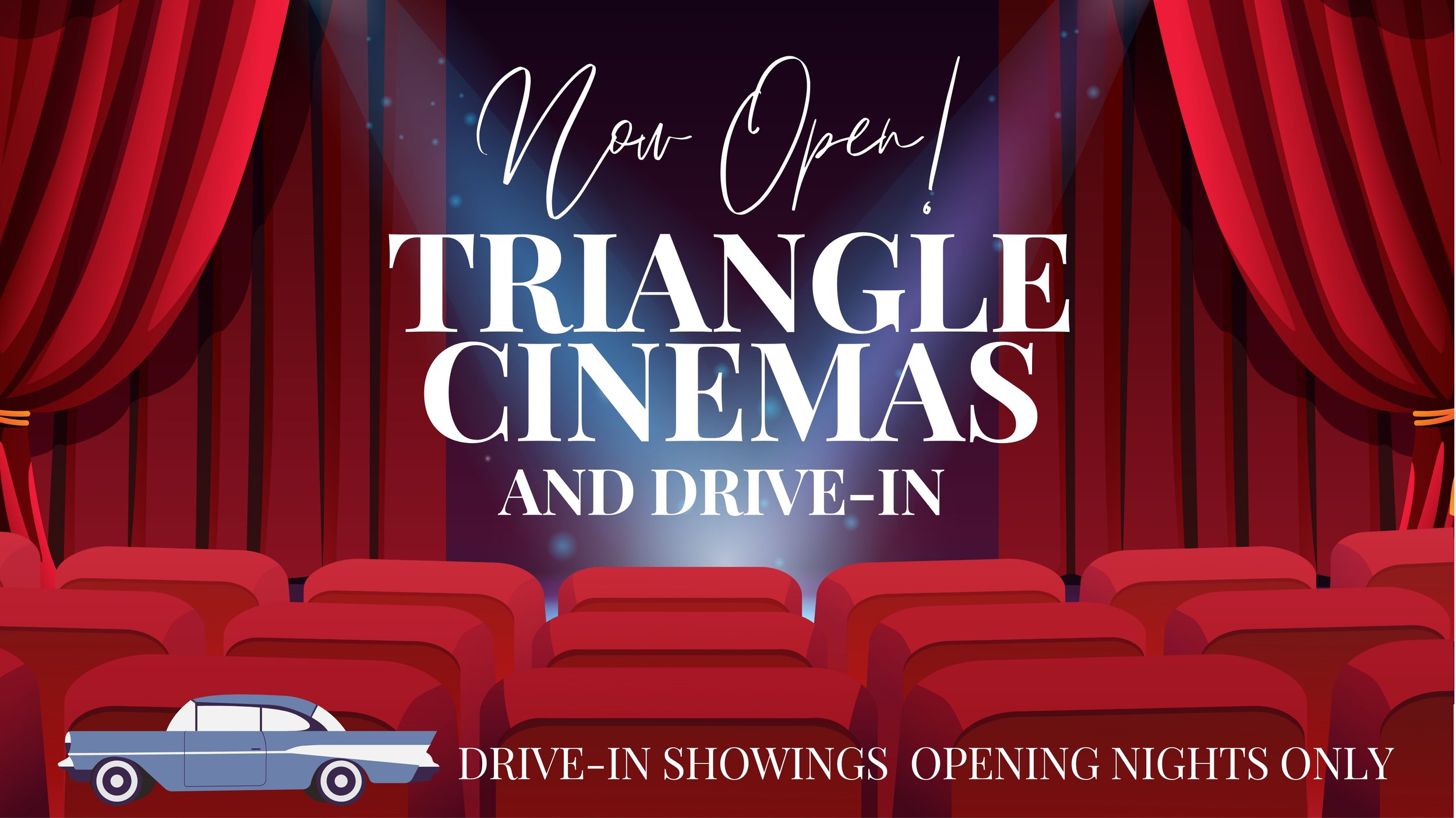The image is an advertisement for a newly opened drive-in theater, Triangle Cinemas and Drive-In. It features a dramatic graphic with a stage set up. There are three rows of red animated chairs, accentuated by long red curtains that are pulled to the side, revealing a part of the stage. In this opening, stylized white script reads, "Now Open! Triangle Cinemas and Drive-In." Below the text, an iconic retro blue car from the 1950s is prominently displayed, alongside text that announces, "Drive-In Showings Opening Nights Only." The overall color scheme combines dramatic dark red and navy blue tones, with all fonts in white, giving a nostalgic yet exciting feel.